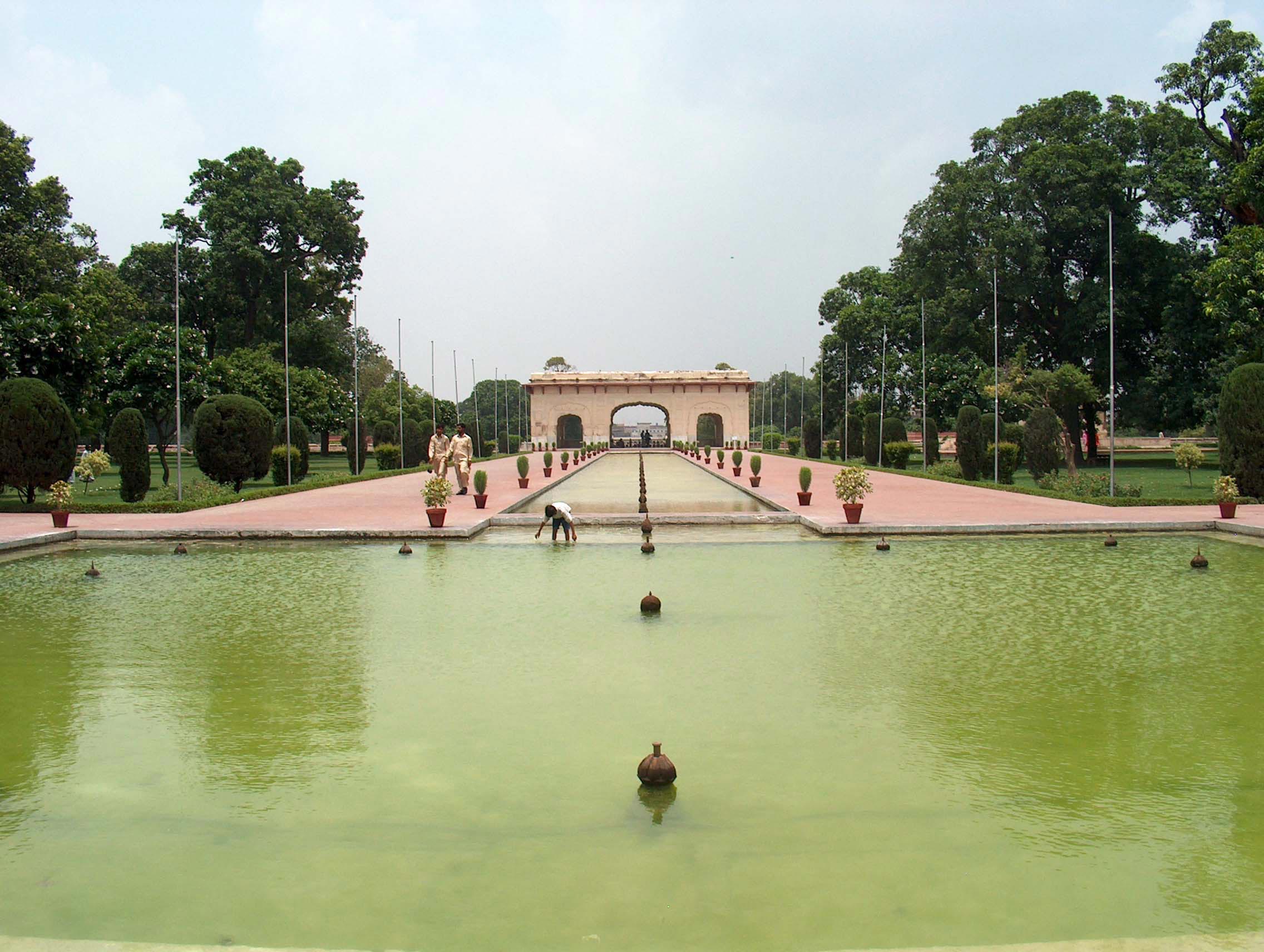This photograph captures a serene and detailed landscape dominated by an artificial, T-shaped reflecting pool filled with green water, suggesting it hasn't been chemically treated. The pool, which begins as a large square in the foreground and extends into a long, narrower strip, is bordered by a wide, pink brick walkway that runs from the left to the right of the image and recedes into the distance. In the middle of the pool, about halfway back, stands a child, while along the walkways, a couple of African-American individuals in gold clothing stroll leisurely.

Flanking the walkways are potted plants featuring cacti, bushes, and dark green trees. Numerous flagpoles or light fixtures line the path, enhancing the structured aesthetic. Interspersed within the water are several large, round pottery-like objects with small openings on top, possibly serving as decorative elements or lights. The scene culminates in a set of tan stone archways at the far end of the pool, featuring two smaller doorways for pedestrians and a grand central archway through which the water might flow, lending an air of architectural elegance to this tranquil outdoor space.